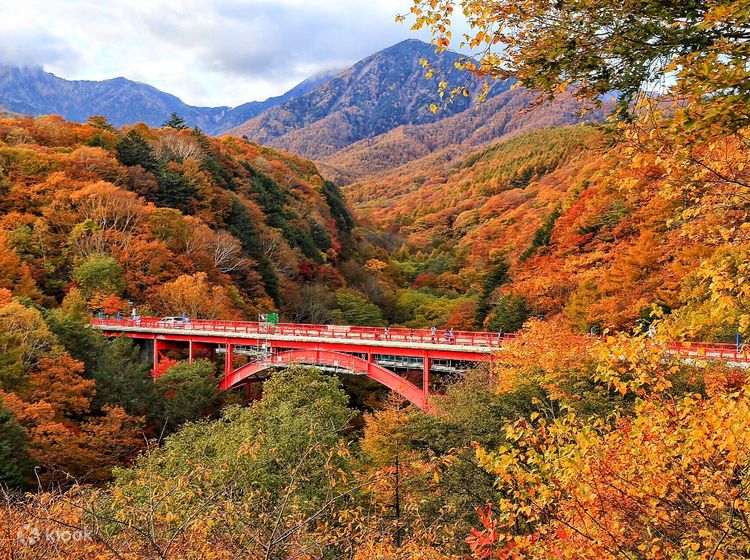This photograph appears to be an old-aged image from possibly the 70s or 80s, capturing a beautiful autumn landscape during the day. The scene is set in a valley surrounded by hills and mountains that are adorned with colorful fall foliage in shades of green, yellow, orange, and red. Stretching from one hill to the other across the valley is a striking red metal bridge with a distinctive arch underneath. The bridge accommodates both pedestrians and vehicles, with visible people walking and a car having recently crossed. The sky in the background features light blue patches with some fog, and a hint of water can be seen in the bottom left corner of the photo. In that same corner, there's a faint stamp, possibly reading "Kayak Book," indicating the manufacturer. The overall composition is framed with detailed brush and greenery, emphasizing the picturesque scenery of the season.